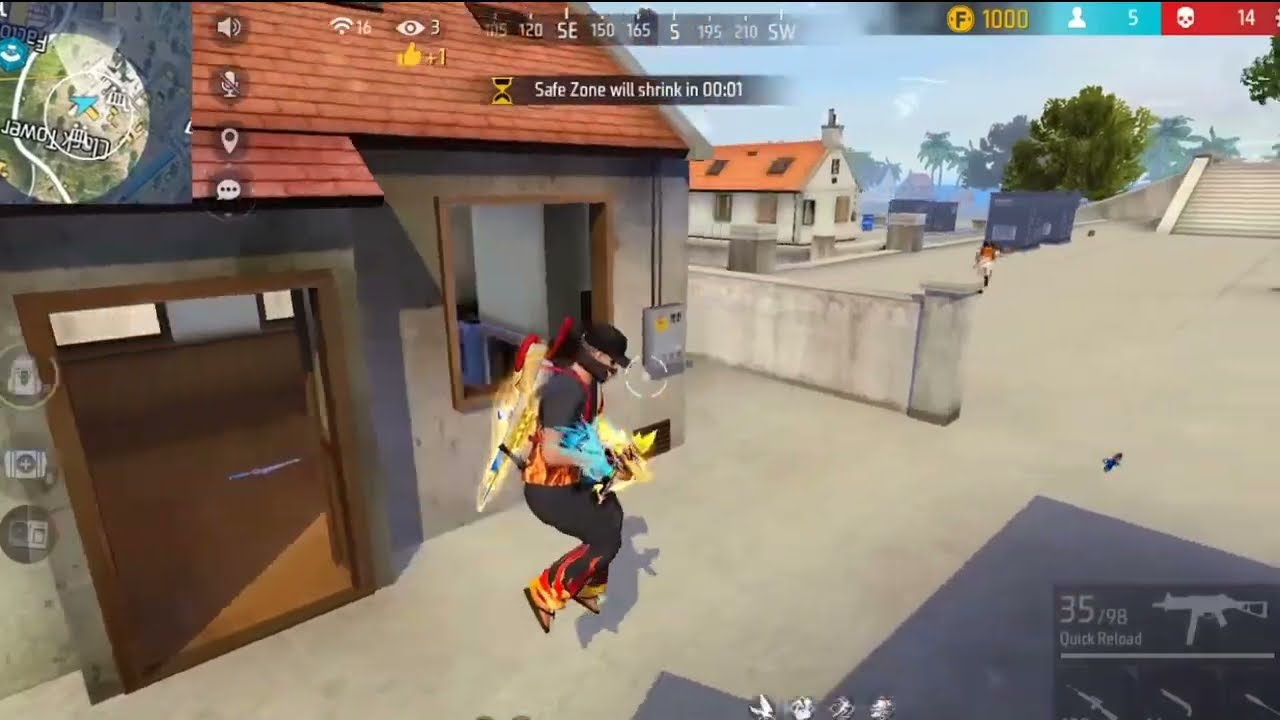In this detailed screenshot from a video game, a character is visibly jumping or possibly using a jet pack to lift off the ground. He is dressed in black pants and a black shirt, both adorned with flames at their bottoms, accessorized with flip flops. The character's face is partially covered with a gator, and he wears a black baseball cap. Strapped to his back is a glowing orange weapon, likely a gun. To his left stands a concrete house with an orange roof and a small wooden door. In the background, there is another indistinct character near a larger concrete building, possibly a church with a distinct figure on top. This building features a large stairway leading up to a plaza. The scene includes a concrete walkway with some trees and an open sky visible. In the right bottom corner of the game interface, there’s an indicator displaying "35/98" alongside a quick reload icon of a gun.